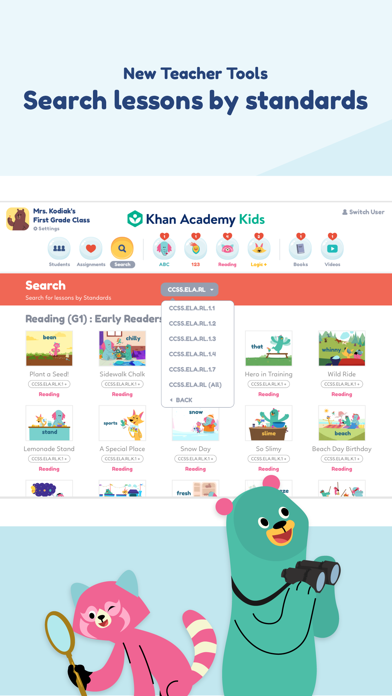This promotional graphic for Khan Academy Kids introduces new teacher tools that facilitate searching for lessons by standards. The graphic features a light blue background at the top, with the text "New Teacher Tools and Search Lessons by Standards" in a dark blue font. 

Beneath the header, the interface of Khan Academy Kids is prominently displayed, showcasing a user's dashboard for Ms. Kodiak's first-grade class. The dashboard features a bear icon representing the user, alongside options for switching users located at the top right. Navigation icons are displayed, including categories such as Students, Assignments, Classes, ABC123, Reading, Logic, Books, and Videos. 

A red-highlighted search bar allows teachers to search for lessons by standards. A drop-down menu lists various standards, including codes like CCSSELARL.1.1 and 1.2. The search results below the menu feature reading lessons for first-grade early readers, displayed as colorful lesson cards. Each card includes a small image and a label with a standard code.

Some example title cards include "Plant a Seed," "Snow Day," "Here When Training," "Beach Day," "So Shiny," and "Birthday." These cards, designed with young learners in mind, are vibrant and mascot-themed, featuring friendly characters such as a pink cat-raccoon hybrid and a blue bear, making the interface engaging and accessible for children.